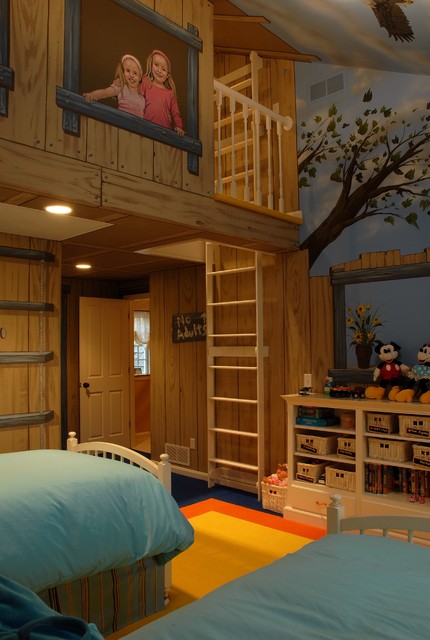The image portrays a charming and spacious children's bedroom, likely in a farm-style home, characterized by blonde wood paneling. The foreground features two twin beds with light blue sheets and white wooden bed frames, positioned next to each other. In front of the beds stands an open-faced white dresser adorned with numerous wicker baskets and an old Mickey and Minnie stuffed animal on top. The room's decor includes a vibrant mural of flowers, a tree, and a blue sky painted on the wall. 

To the left of the room, there is an indoor treehouse structure that extends up to a second-floor loft area, accessed by two ladders—one wooden and one rope. Adjacent to the treehouse, a painted photograph of two smiling girls, the older girl in a dark pink shirt and the younger in a light pink shirt, is displayed. A "No Adults" sign humorously hangs to the right of the room's open door, which opens into a hallway. This delightful space appears not only functional but also imaginative, making it an ideal bedroom and play area for the two children.